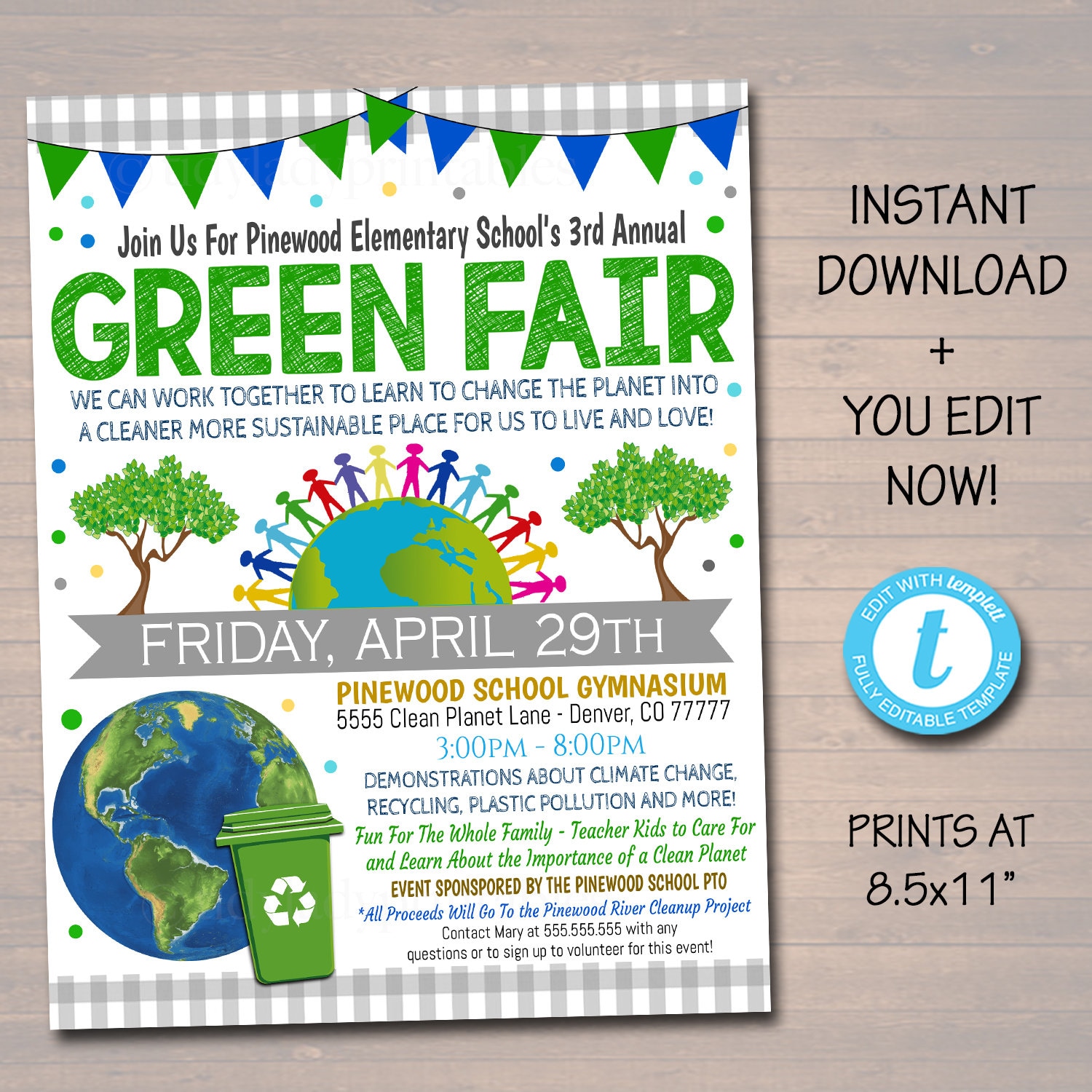The image is a computer-generated flyer for Pinewood Elementary School's third annual Green Fair. The background of the flyer includes a wooden-paneled design with a white and gray striped pattern appearing at the top and bottom of the image. Green and blue triangular banners drape across the top of the flyer, adding a festive touch.

The main body of the flyer, set against a white backdrop, features black lettering that invites the viewer to "Join us for Pinewood Elementary School's 3rd Annual Green Fair" with the words "Green Fair" prominently displayed in bold green letters. Centrally located on the flyer is a vibrant depiction of a globe surrounded by multicolored figures—yellow, blue, light blue, green, red, and purple—holding hands, symbolizing unity and environmental stewardship. Flanking this central image, two green trees add to the eco-friendly theme.

Below this main graphic is a gray banner that provides the event's date: "Friday, April 29th." In the bottom left corner, there is an additional image of Earth, showing blue oceans and green continents, alongside a green recycling bin bearing the recycling symbol. To the right of the poster, there is black text mentioning an instant download and a blue button labeled "Edit with template," promoting an editable version of the flyer. The overall design is inviting, emphasizing the theme of coming together to promote sustainability at Pinewood Elementary School's annual Green Fair.